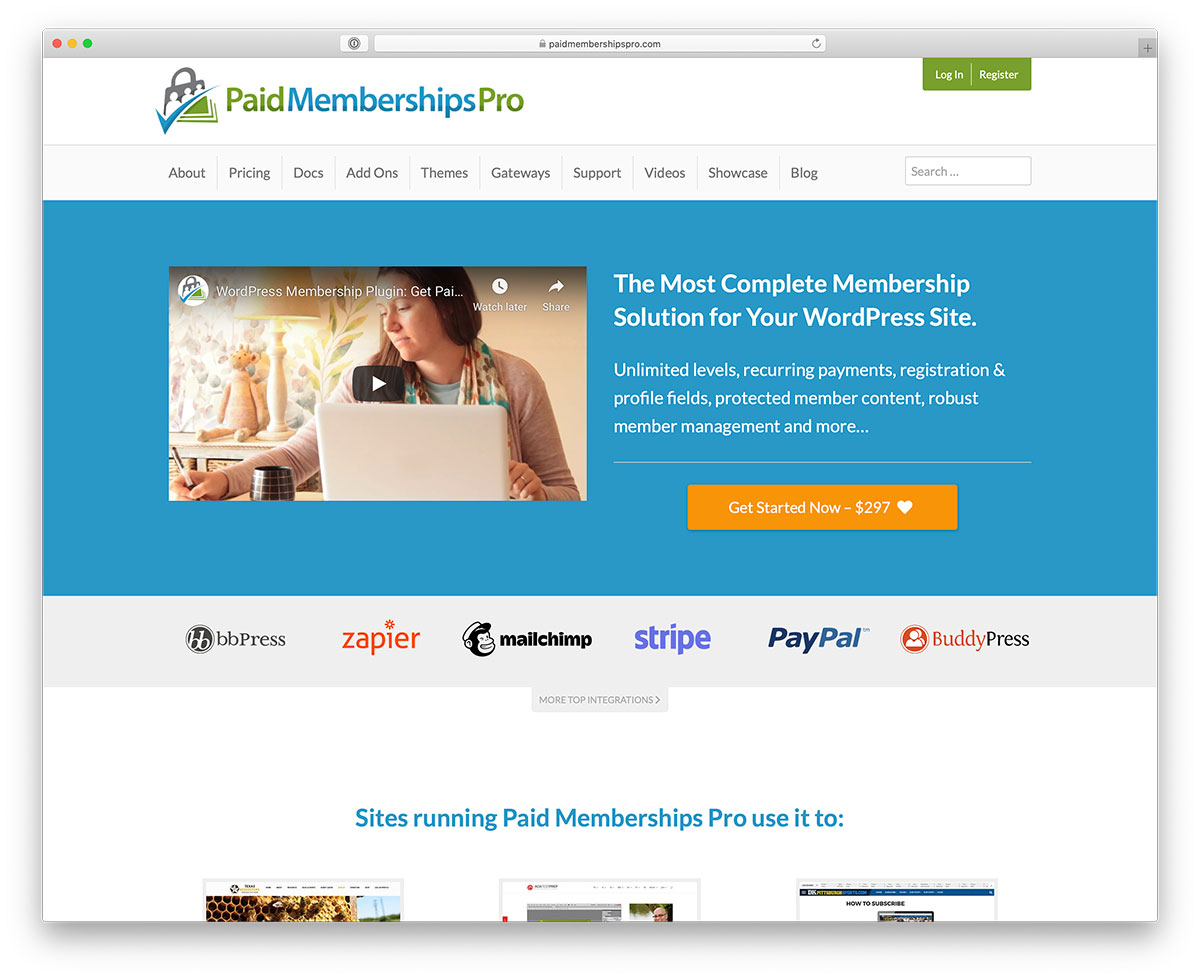The image features a comprehensive promotional banner for Paid Memberships Pro, a WordPress membership plugin. 

**Top Section:**
- **Top Left:** Prominently displays the "Paid Memberships Pro" logo.
- **Top Right:** Options to "Login" and "Register," emphasizing user account access.
  
**Navigation Menu (Below the Login/Register Options):**
- A sequence of navigation links listed as: "About," "Pricing," "Docs," "Add-ons," "Themes," "Gateways," "Support," "Videos," and "Showcase."
  
**Search Feature:**
- A Bing search box is included, facilitating quick search functionality.

**Main Content (Central Area):**
- The background is primarily blue, featuring a woman using a laptop, suggesting user interaction with the software.
- On a table behind her, there is a lamp and a doll, adding a homely touch to the setting.
  
**Key Marketing Text (Right of the Woman):**
- A headline stating, **"The Most Complete Membership Solution for Your WordPress Site."**
- Bullet points highlighting key features:
  - Unlimited levels
  - Recurring payments
  - Registration and profile fields
  - Protected member content
  - Robust member management
  - And more.
- A call-to-action button with the text **"Get started now for $297."**
- An accompanying white heart graphic.

**Additional Information (Bottom Section):**
- Logos and mentions of compatible services: "BB Press," "Zapier," "Mailchimp," "Stripe," "PayPal," and "BuddyPress."
- A note stating, "Sites Running Paid Memberships Pro, Use It 2," indicating extensive use of the plugin.
- The display includes three partial screenshots of websites utilizing the plugin, although they are cut off at the bottom edge.

This detailed description encapsulates the promotional content and layout effectively, offering clear insight into the visual and textual elements presented in the image.